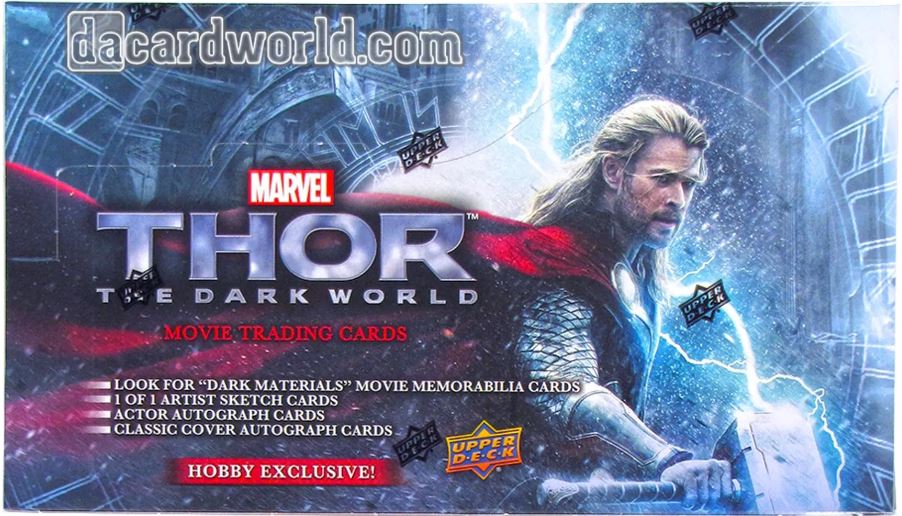This is an advertisement poster for Upper Deck's movie trading cards from the film "Thor: The Dark World." Prominently featured is the superhero Thor, grasping his iconic hammer, Mjolnir, with his red cape flowing behind him. Lightning bolts emanate from the hammer, adding dramatic effect to the scene. Thor stands in front of a giant, blue-colored circular machine, suggesting a high-tech setting. The top left corner of the poster displays "dacardworld.com," while text below to the left of Thor reads, "Marvel Thor The Dark World Movie Trading Cards." The poster details the exclusive content offered in the hobby boxes, including dark materials, movie memorabilia cards, one-of-one artist sketch cards, actor autograph cards, and classic cover autograph cards. Upper Deck's quality seals are present, reinforcing the authenticity of the product. The overall imagery emphasizes Thor’s elemental power and his traditional outfit, further enhancing the heroic and electrifying theme of the advertisement.